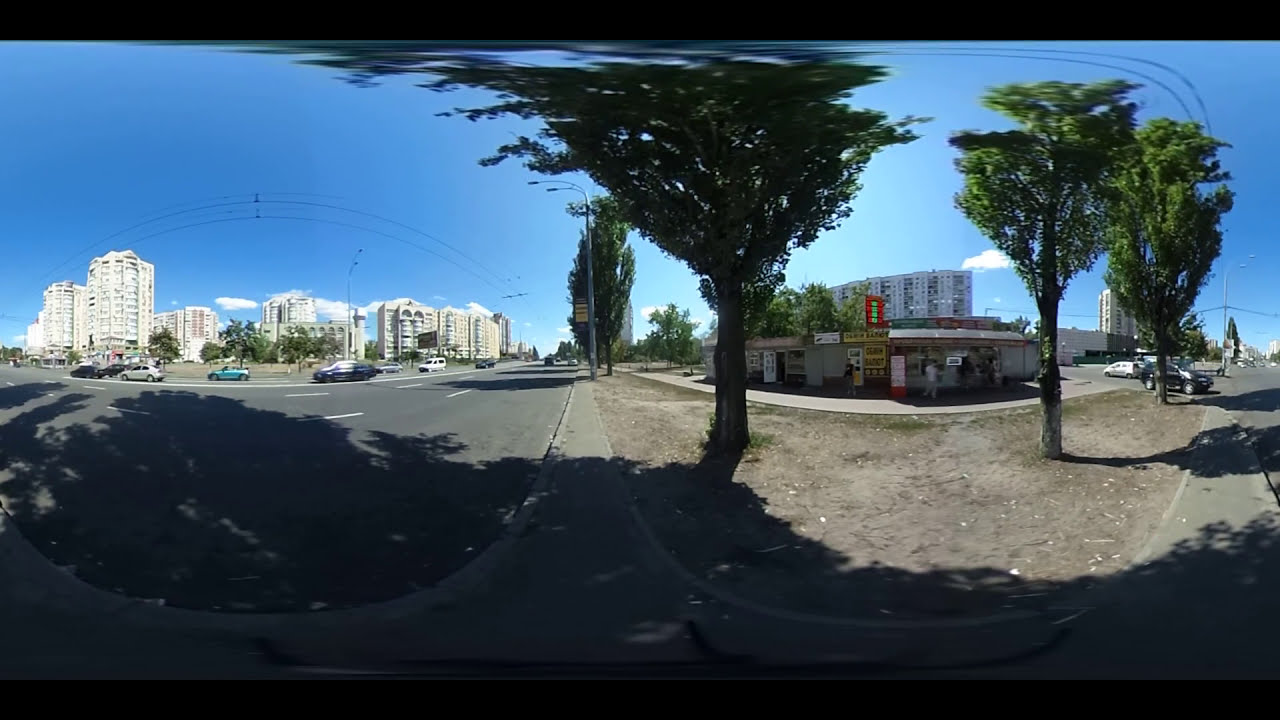This image is a warped cityscape panorama captured with a fisheye lens, giving it a distinctive distorted effect. The scene is set in an urban environment with a prominent, broad cement four-lane highway on the left, carrying about half a dozen cars toward the left side of the frame. Adjacent to the highway is a central sidewalk that ripples and curves outward due to the fisheye distortion, creating a unique U-pattern. The panoramic format reveals a blend of two separate photographs seamlessly combined, accentuating both distant and close perspectives.

On the left side of the image, in the far background, stand multiple off-white and beige high-rise apartment buildings, accompanied by green trees that seem part of the distant sidewalk. Electric cables are visibly intertwined above, particularly to the center-left, standing out against a backdrop of a mostly blue, partly cloudy sky.

The right side of the image features a single-story convenience store with yellow and white signage, set slightly apart by a parking lot where a few cars are stationed. Near the store, you can also see additional trees—their branches adorned with vibrant green leaves. The foreground is marked by a dirt patch leading up to the sidewalk, further enhancing the feeling of depth. Overall, the photographic style is representational, capturing the realism of the urban setting with detailed and panoramic precision.